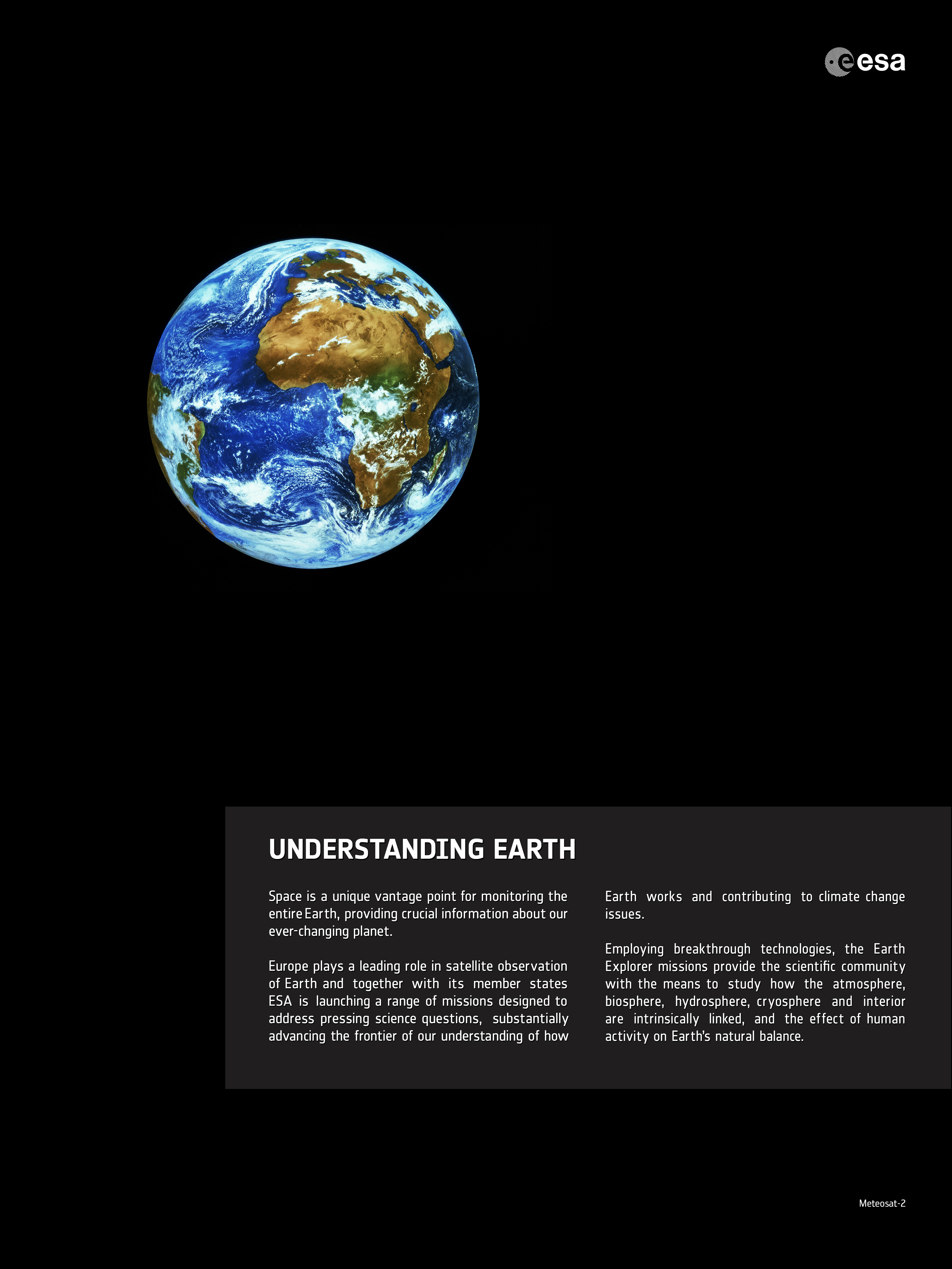This screenshot, captured in portrait mode, features a strikingly minimalistic black background. In the top right corner, the European Space Agency (ESA) logo is prominently displayed. Centrally, an exquisite image of Earth is highlighted, with the globe's focus on the African continent and the surrounding vast oceans adorned with swirling white patterns, indicative of cloud formations.

Positioned in the bottom right corner is the text "METEOSAT-2," which identifies the specific satellite source of the imagery. Slightly below the center and toward the right, a content block succinctly conveys the following message: 

"Understanding Earth. Space is a unique vantage point for monitoring the entire Earth, providing crucial information about our ever-changing planet. Europe plays a leading role in satellite observation of Earth, and together with its member states, ESA is launching a range of missions designed to address pressing science questions, substantially advancing the frontier of our understanding of how Earth works and contributing to climate change issues. Employing breakthrough technologies, the Earth Explorer missions provide the scientific community with the means to study how the atmosphere, biosphere, hydrosphere, cryosphere, and interior are intrinsically linked and the effect of human activities on Earth's natural balance."

This image captures both the beauty of our planet from space and the vital role Esa plays in advancing our knowledge and addressing global environmental challenges.